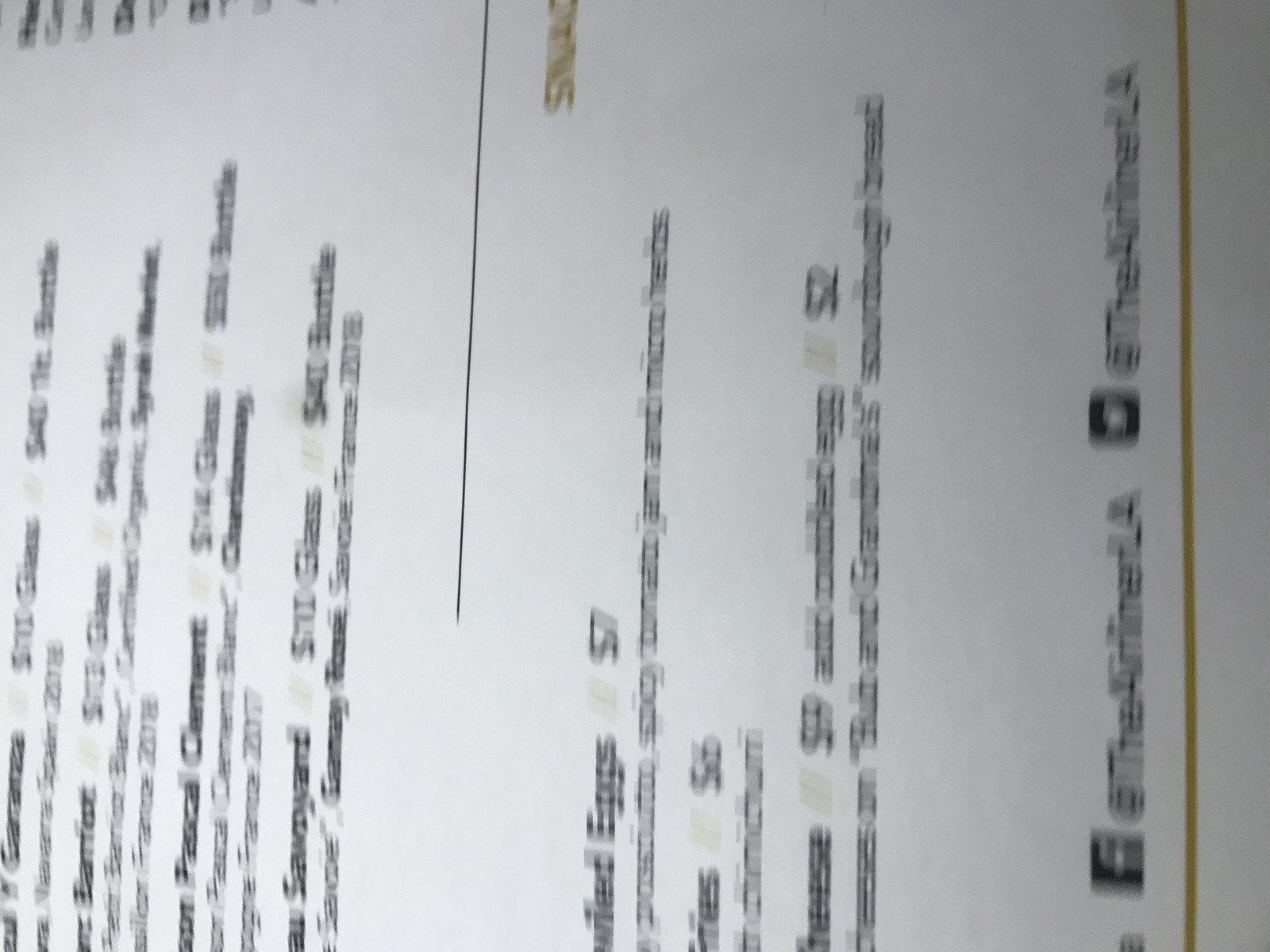A picture captures a menu displayed on its side, requiring a tilt to read it upright. The menu is divided by a central vertical line and another gold-hued vertical line on the right. Alongside the central vertical line, some of the text is highlighted in gold. The majority of the text is in black, featuring bold item names followed by descriptions and corresponding prices. Adjacent to each price, there's a faint tan notation, adding a subtle touch of detail.